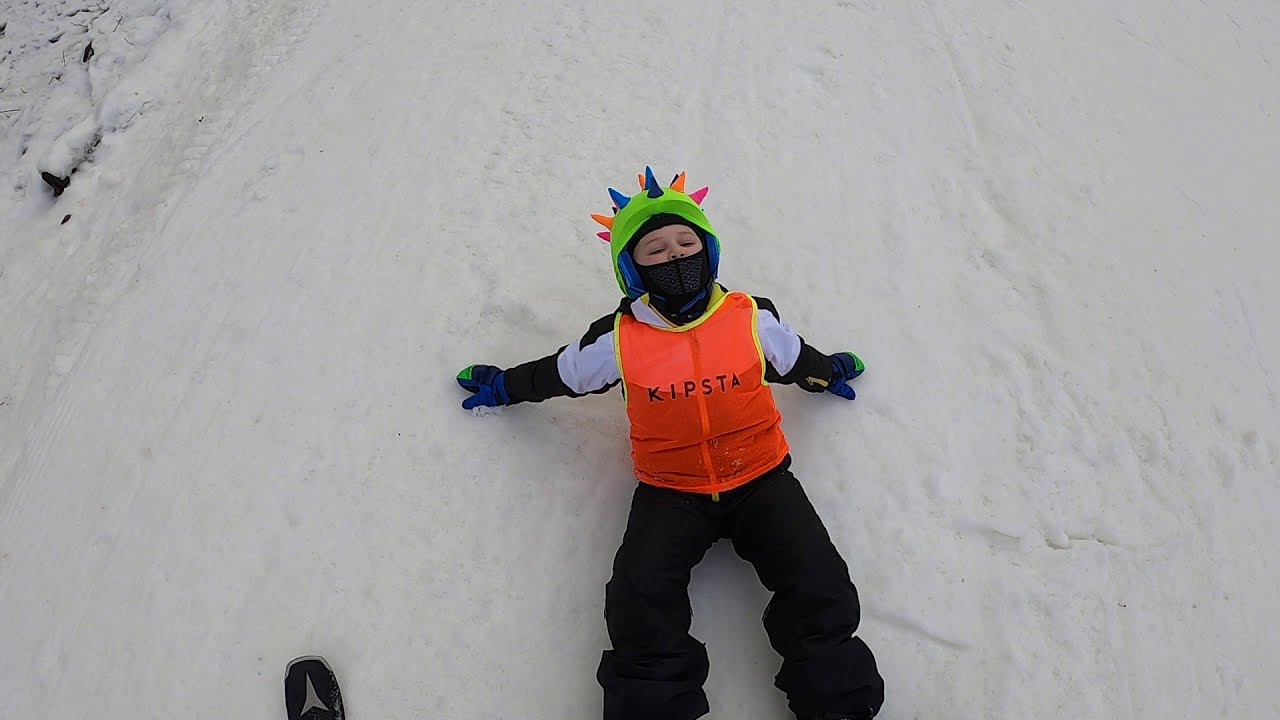The image shows a young boy relaxing in the snow, taken from above. He is seated with his knees bent, leaning back on his arms, his head tilted upwards. He is dressed in a black and white snowsuit topped with a bright orange vest that says "Kipsta" in black text. He wears a ski mask and an eye-catching green helmet adorned with multicolored spikes that resemble a dinosaur. His gloves are blue and green, adding to the vibrant ensemble. In the bottom left corner of the frame, the black and gray shoe of another person, likely the photographer, is visible. The surrounding scenery is predominantly snow-covered, with a few scattered rocks in the upper left corner, giving the impression of overcast weather. The boy appears to be taking a break, enjoying a moment of rest in the snow.